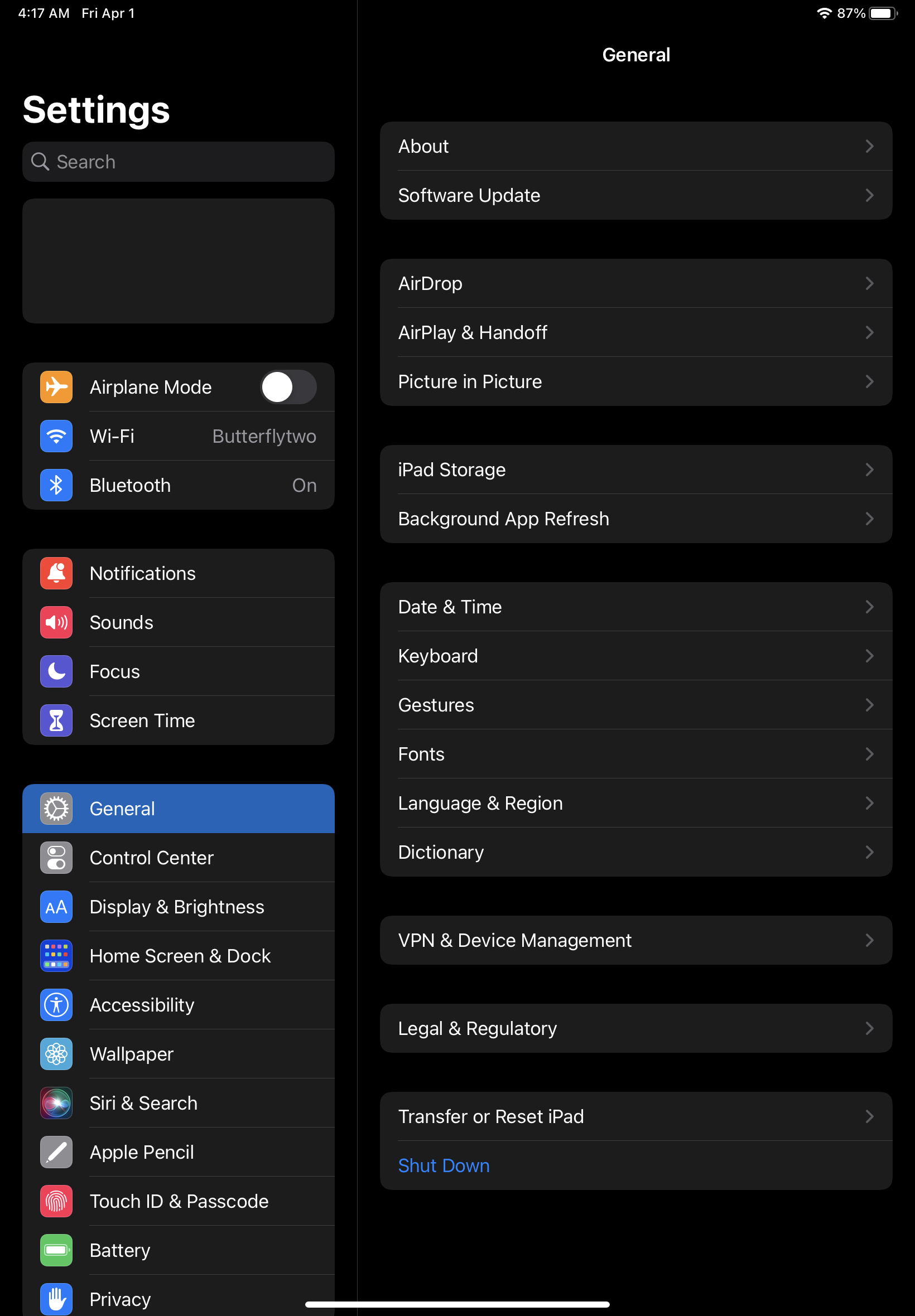This image, categorized under the "website" section, depicts a smartphone screen displaying its settings menu. Captured at 4:17 a.m. on April 1st, the timing hints at it perhaps not being the best moment for adjustments. At the top of the screen, a "Settings" header is prominently displayed, along with a search bar for easy navigation.

Visible options include:
- **Airplane Mode**: Currently toggled off.
- **Wi-Fi**: Connected to a network named "Butterfly 2".
- **Bluetooth**: Activated.

Following these, additional settings are listed, such as:
- **Notifications**
- **Sounds**
- **Focus**
- **Screen Time**

The "General" category is highlighted, revealing a plethora of options:
- About
- Software Update
- AirDrop
- AirPlay & Handoff
- Picture-in-Picture
- iPad Storage
- Background App Refresh
- Date & Time
- Keyboard
- Gestures
- Fonts
- Language & Region (initially misread as "language and religion")
- Dictionary
- VPN & Device Management
- Legal & Regulatory
- Transfer or Reset
- Shut Down

Adjacent to "General", other categories include:
- Control Center
- Display & Brightness
- Home Screen & Dock
- Accessibility
- Wallpaper
- Siri & Search
- Apple Pencil
- Touch ID & Passcode

The image meticulously captures the array of customizable settings available on the phone, portraying the depth and variety of options users can configure.